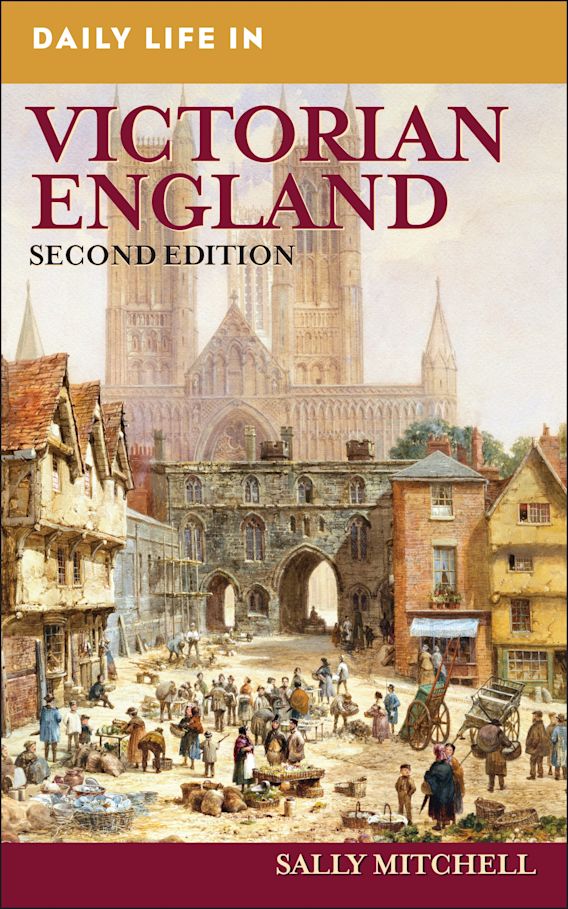This is a detailed photograph of the book cover for "Daily Life in Victorian England, Second Edition" by Sally Mitchell. The title "Daily Life in" is left-justified in white text against an amber-brown background. "Victorian England" is prominently displayed in a serif font, all caps, on a goldish background, while "Second Edition" appears in smaller black font below it. The bottom section features the author's name in white, all caps, on a burgundy background.

The main illustration on the cover is a bustling depiction of a Victorian village scene, rich with details. In the center, a large wide dirt street is flanked by various buildings that likely serve as both homes and businesses, distinguishable by their windows and architectural style. To the left, there are houses, and in the middle, a drawbridge is situated. The village is teeming with activity; numerous little figures are shown engaged in different aspects of Victorian life, such as an outdoor open market where people are selling fruits, vegetables, and possibly sacks of grain. Some handheld push carts are either at rest or in use, contributing to the dynamic market atmosphere.

In the background, towering over the village, is a large cathedral or church with several high vertical towers and inlaid glass windows, adding a historical authenticity to the scene. The city appears full of life, with people constructing things, moving in and out of stores, and generally going about their daily routines in this vibrant Victorian setting.